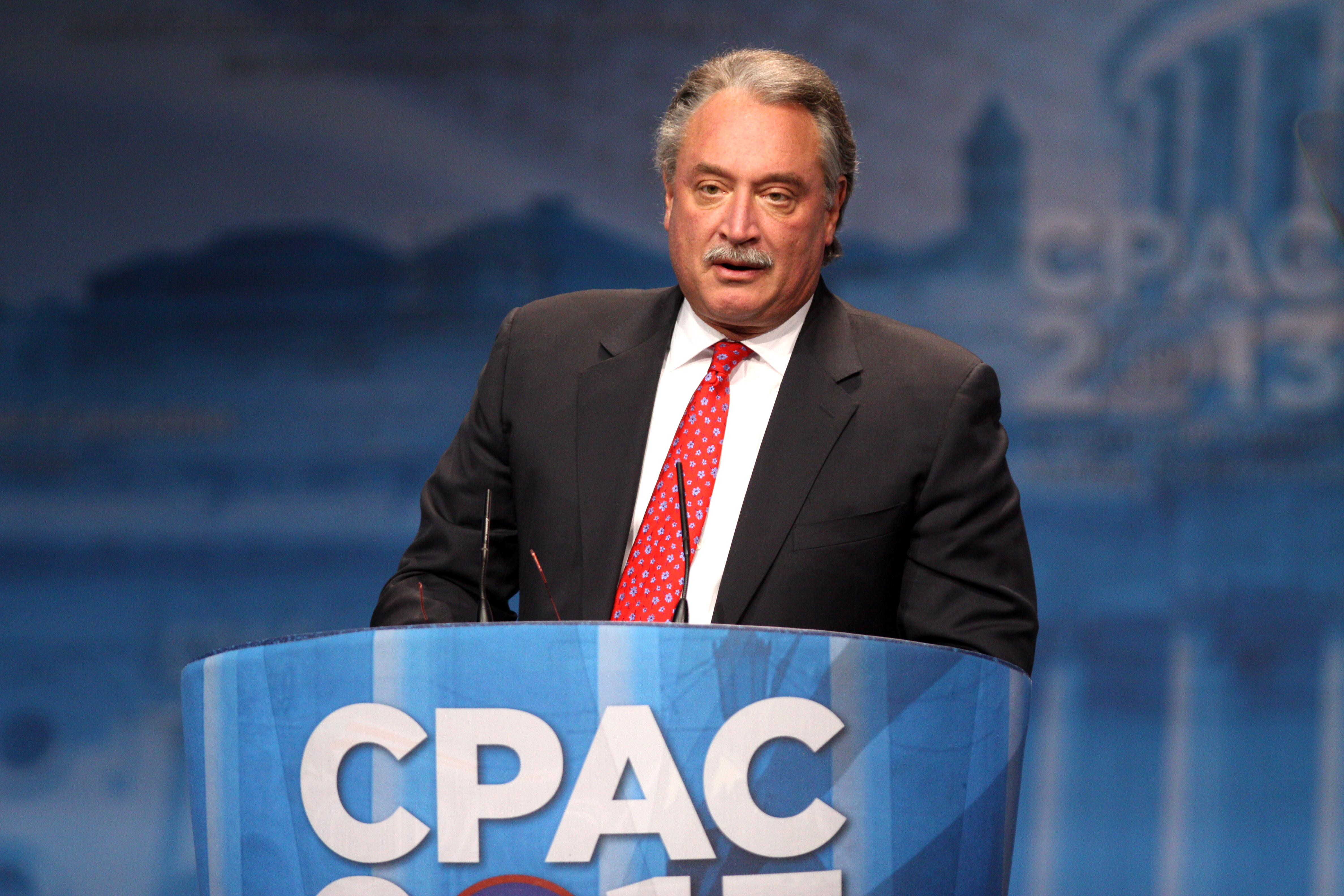A man with gray hair and a gray mustache stands behind a blue, rounded podium that prominently features the letters "CPAC" in large, bold white text. He is dressed in a dark suit jacket, a white shirt, and a red tie with blue dots. Small microphones point towards him from the podium. The background is a blurred blue scene with images of monuments and buildings, likely indicative of Washington, D.C. In white text on the upper right side of the background, partially legible, it reads "CPAC 2013."